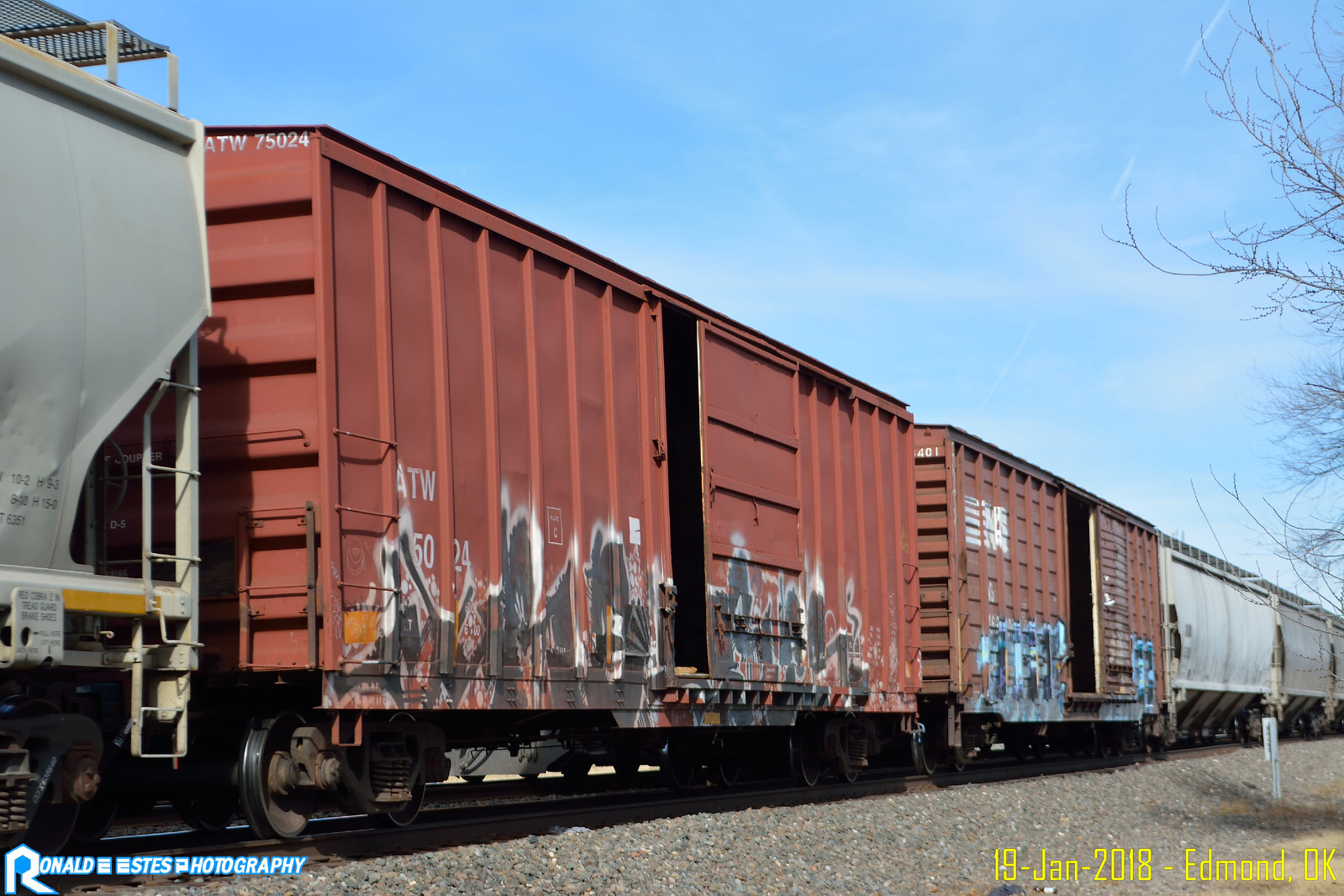This photograph captures a freight train situated in Edmond, Oklahoma, taken on January 19th, 2018, by Ronald Estes Photography, as indicated by the watermark in the bottom left corner and the date and location in the bottom right. The train extends from the left side to the lower right corner, creating a visual perspective that makes the railway cars appear progressively smaller as they recede into the distance. 

From left to right, the first visible car is a grayish engine marked with "102H93-940H15-0" and is equipped with a ladder. Following this, there's a burnt reddish-orange cargo car labeled "ATW75024," its sliding door slightly ajar, adorned with graffiti in black and white spray paint. This is succeeded by another reddish-orange cargo car, also with a partially open door, featuring graffiti in white, blue, and black. Farther along, there are two additional white cargo cars, unmarked by graffiti, that fade more into the background due to the perspective.

Above the train, the sky is a clear blue with a few scattered clouds, and a tree with bare branches appears on the far right, hinting at the winter season. This detailed capture not only highlights the train's journey but also the urban art that accompanies it.